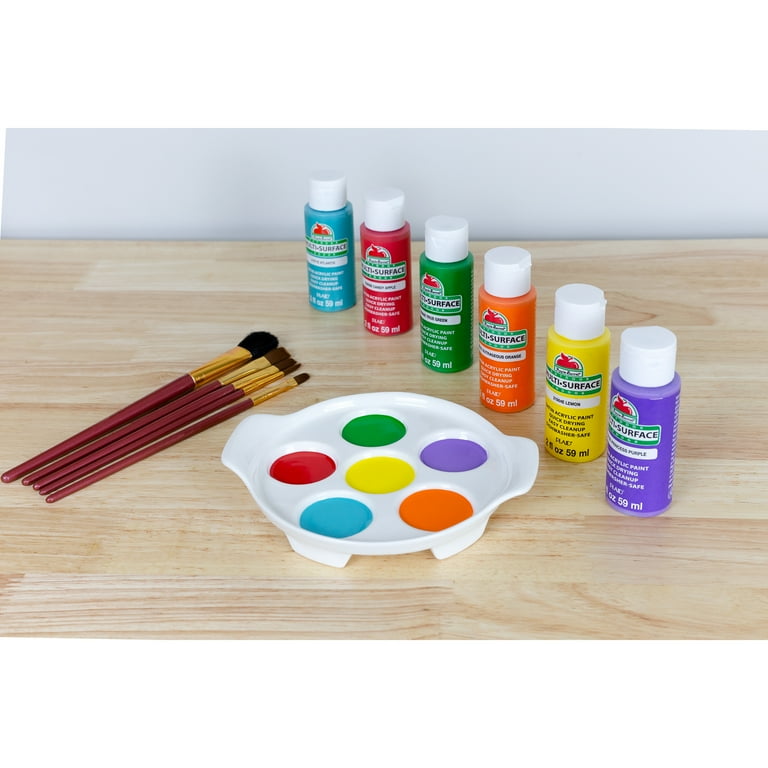On a light brown table, a variety of art supplies are neatly arranged, creating a well-organized palette for creativity. Six bottles of acrylic paint with white caps are positioned diagonally on the right side of the table, descending from the top of the image. The colors of the bottles from top to bottom are turquoise, red, green, orange, yellow, and purple. In the middle of the table, in front of the paint bottles, there is a white paint palette holding six different colors. The top row of the palette displays red, green, and purple from left to right; the center holds yellow, and the bottom row features blue and orange from left to right. To the left side of the table lies an array of five paint brushes with brown handles, varying in size and meticulously lined up, ready for use.